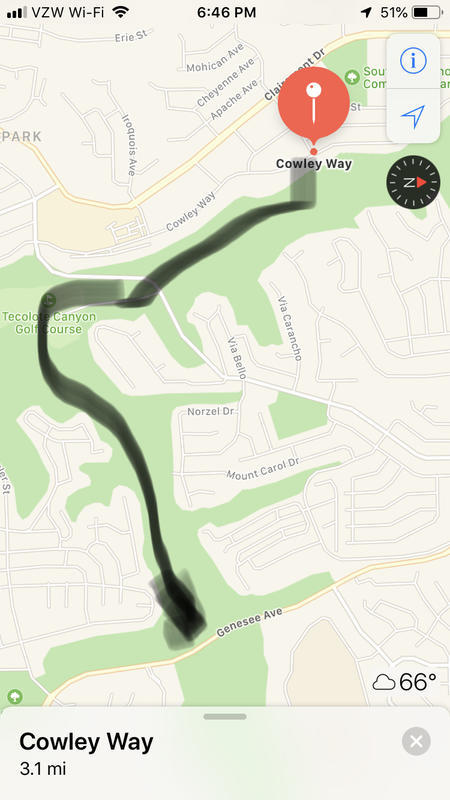Screenshot of a map application on a cell phone, likely an iPhone, displaying details for a hike to Cowley Way. The interface includes a pale grey status bar at the top showing signal strength, Wi-Fi provider, current time, and battery percentage. The map features typical color coding with grey and green areas for terrain, and yellow or white lines for roads. A pin marks Cowley Way, which is 3.1 miles from the starting point. The user has used the edit function to draw a rough and wide black line indicating the hiking route, which starts on an avenue, traverses through a green section, and follows the park's length to reach Cowley Way. A temperature reading of 66 degrees is visible in the bottom right corner, and the distance to Cowley Way is displayed in a grey block at the bottom with a close symbol.